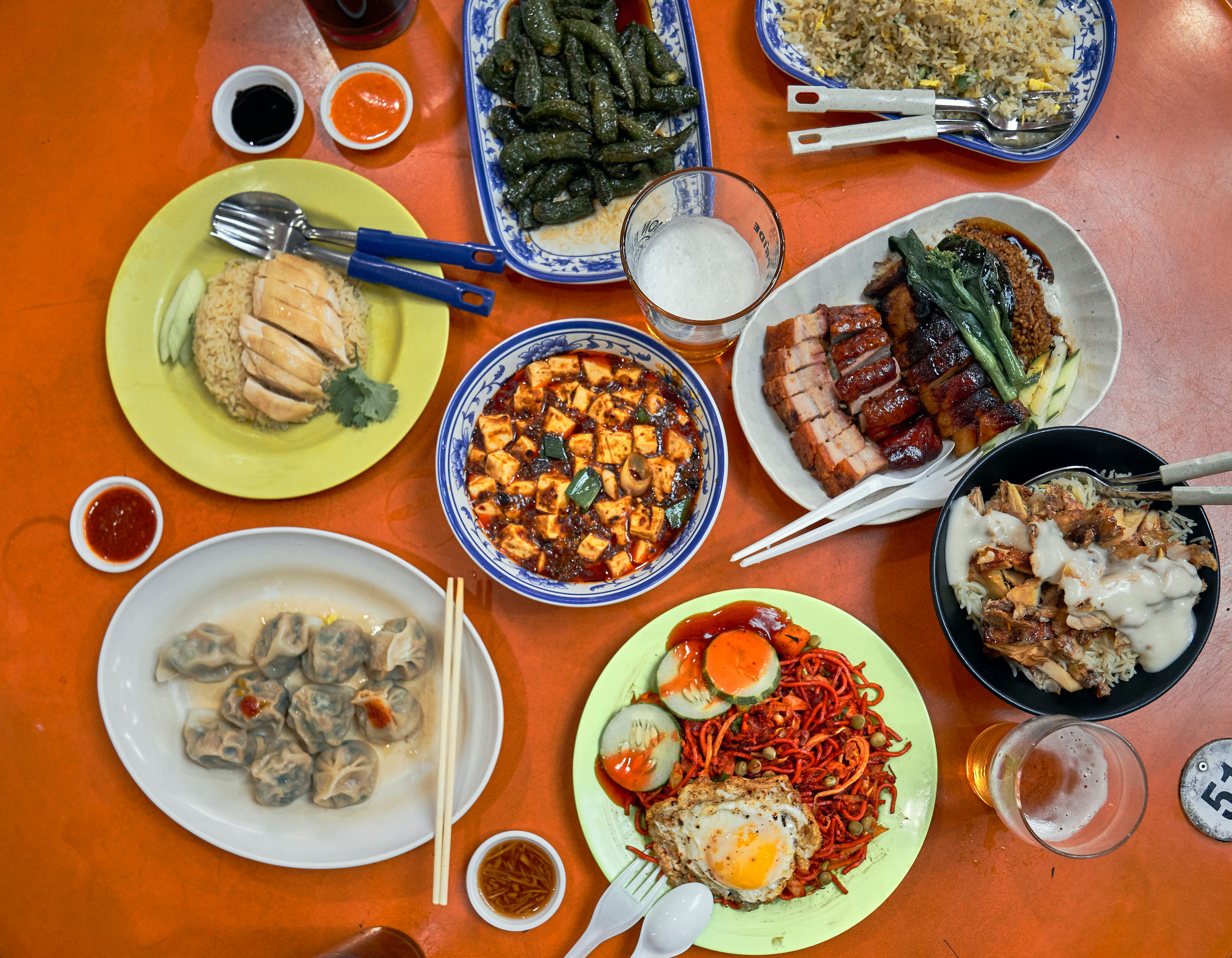This close-up photo captures an abundant and diverse spread of food displayed on an orange table with a red-orange tablecloth, showcasing a feast that appears untouched and ready to be served. Central to the table is an enticing variety of dishes:

In the lower-left corner, a plate of spicy dumplings garnished with red spices sits next to a red dipping sauce and a chili sauce. Above that, a chicken dish rests on a circular pancake of rice. 

Directly in the center are chickpeas paired with more chicken, surrounded by a large rack of ribs that vary in color and are garnished and sauced to perfection. Below the ribs, a refreshing cucumber and radish salad provides a vibrant contrast.

On the right side, a detailed lamb dish is presented next to a dark, meaty soup holding light brown chunks of meat. To accompany the soup, there's a large bowl of mashed potatoes topped with green garnishes and a plate of green beans. Another notable dish nearby contains rice and beans.

Amidst this array, a blue and white rectangular dish is laden with dark leafy greens on a bed of rice, accompanied by a fork and spoon. Adjacent to it, another blue and white dish carries rice mixed with eggs. 

An oval white platter holds grayish lumps of an unspecified dish, contributing to the eclectic mix. Additionally, four small circular dishes of various dipping sauces add to the flavors on offer, while beverages including foaming beer and milk complete the scene. Plastic utensils are placed throughout, ready for the meal to commence.